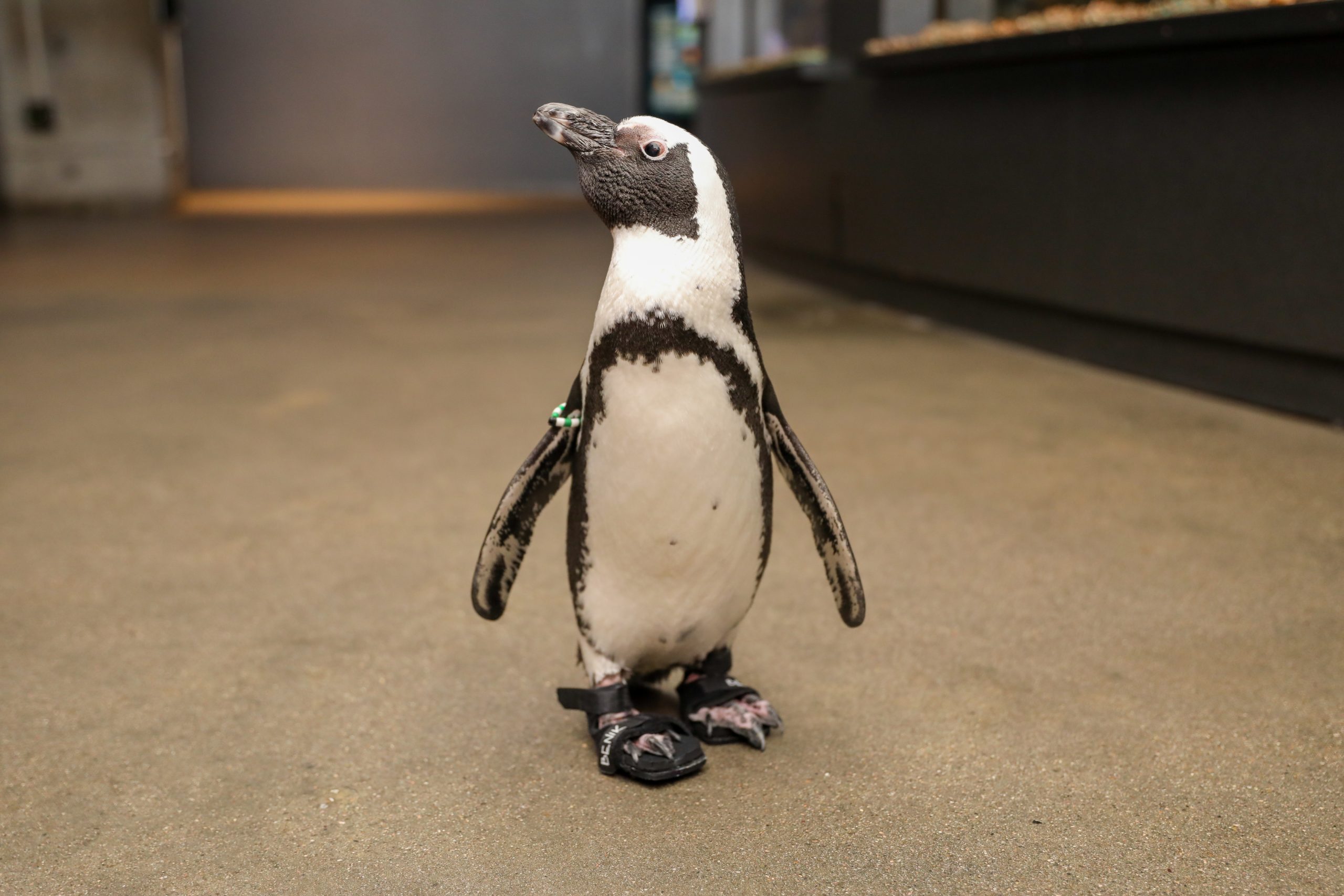In this image, there is a close-up photograph of a small penguin, barely two feet tall, standing on a light, tannish, grainy concrete floor. The penguin has a distinctive appearance with a white body, a white neck, and black markings including a black face, black beak, and a black stripe across its neck. It is wearing black sandals or rubber flip flops on its feet. On its left flipper near the shoulder, it has a beaded bracelet made up of white, green, and possibly black beads, which may be a name tag or number tag. The penguin is looking to the left. In the background, there is a gray wall and a door with light seeping through the bottom, along with a black counter and a square-shaped window on the right side, suggesting the setting is an interior space, possibly a veterinary room.